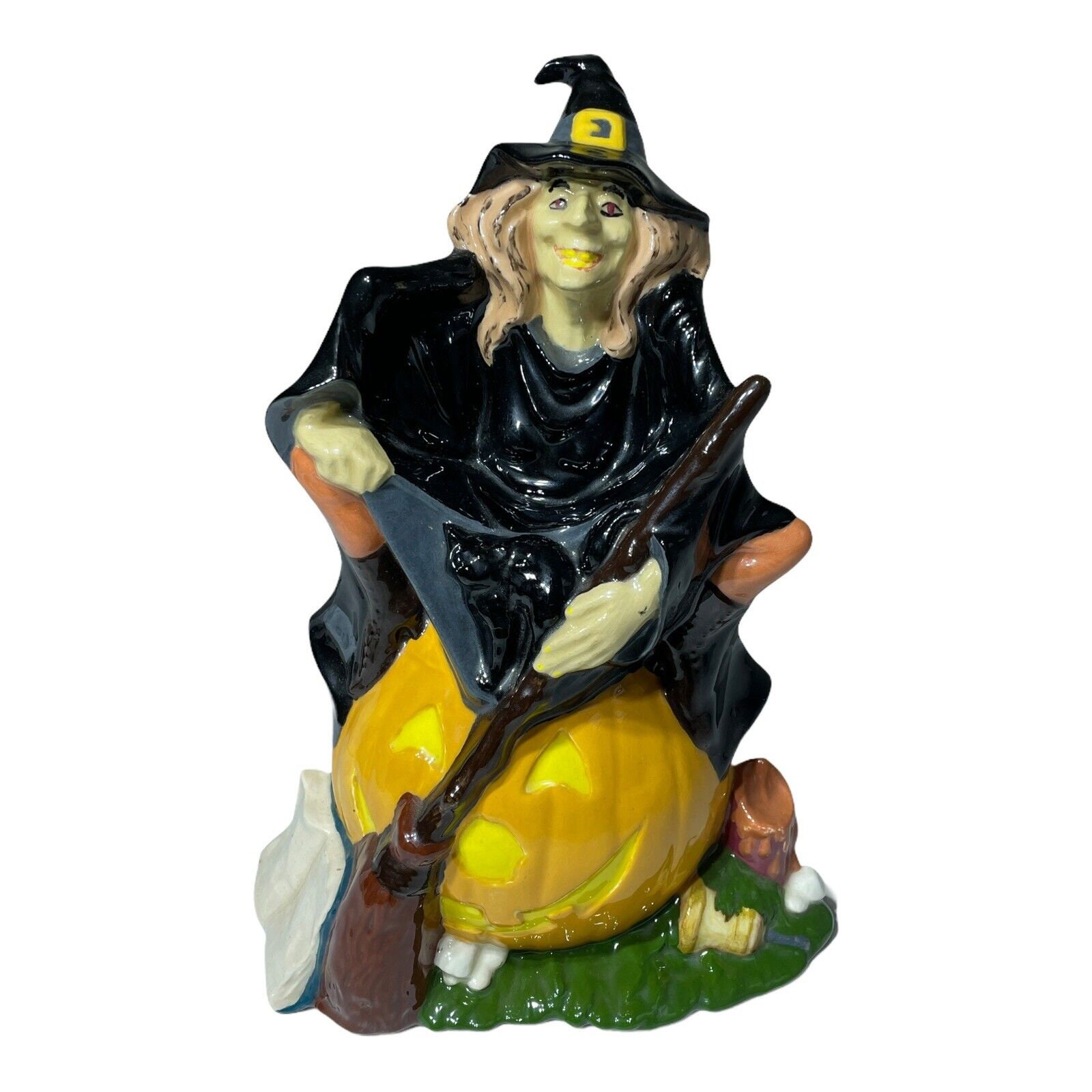This porcelain Halloween decoration depicts a witch figure seated atop an orange jack-o'-lantern. The witch, dressed in traditional black robes, black boots, and a loose-fitting top, is crouching on the pumpkin with a mischievous grin. Her pale greenish-yellow skin and worn appearance give her an aged look, while her long, light brown hair cascades from beneath a black hat, adorned with a blue band and a gold buckle. The witch's face is particularly detailed, showing yellow teeth and buck teeth with a noticeable gap. In her right hand, she firmly grasps a broomstick, the bristles of which are brown, and her left hand is poised as if adjusting her attire.

The jack-o'-lantern she sits on features bright yellow eyes, nose, and a happy smile, giving it a friendly demeanor. Below the pumpkin, a textured green grass base adds to the scene's ambiance, with various small elements scattered about. These include a half-eaten yellow apple core, a white bag, a tree stump, and what appears to be a bell lying on the grass. In addition, a cartoonish dwarf head peeks out from the right side of the pumpkin, enhancing the whimsical nature of the figurine. The overall scene creates a lively and intricate Halloween-themed decoration, blending various small details into a cohesive and charming display.